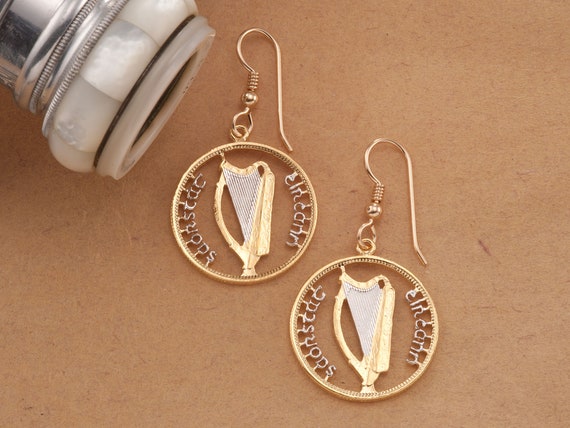In the photograph, two large gold hoop earrings lie elegantly on a brown tabletop. Each earring features a delicate circular outline, with a central gold harp intricately crafted inside the hoop. The strings of the harp are silver, enhancing the overall elegance and contrast within the golden structure. Surrounding the perimeter of each earring is an inscription in what appears to be a foreign language or Greek lettering, adding a layer of mystery and sophistication. The earrings, identical in design, are arranged with one centrally positioned and the other slightly lower and to the right. In the upper left corner of the image, a silver and white object—possibly part of a blow dryer or a jewelry container—intrudes into the frame, suggesting a mundane setting where the earrings might be cleaned or stored. The background is a smooth cream-brown surface that highlights the intricate details and shimmering quality of the earrings, making them especially striking for someone who appreciates or plays the harp.